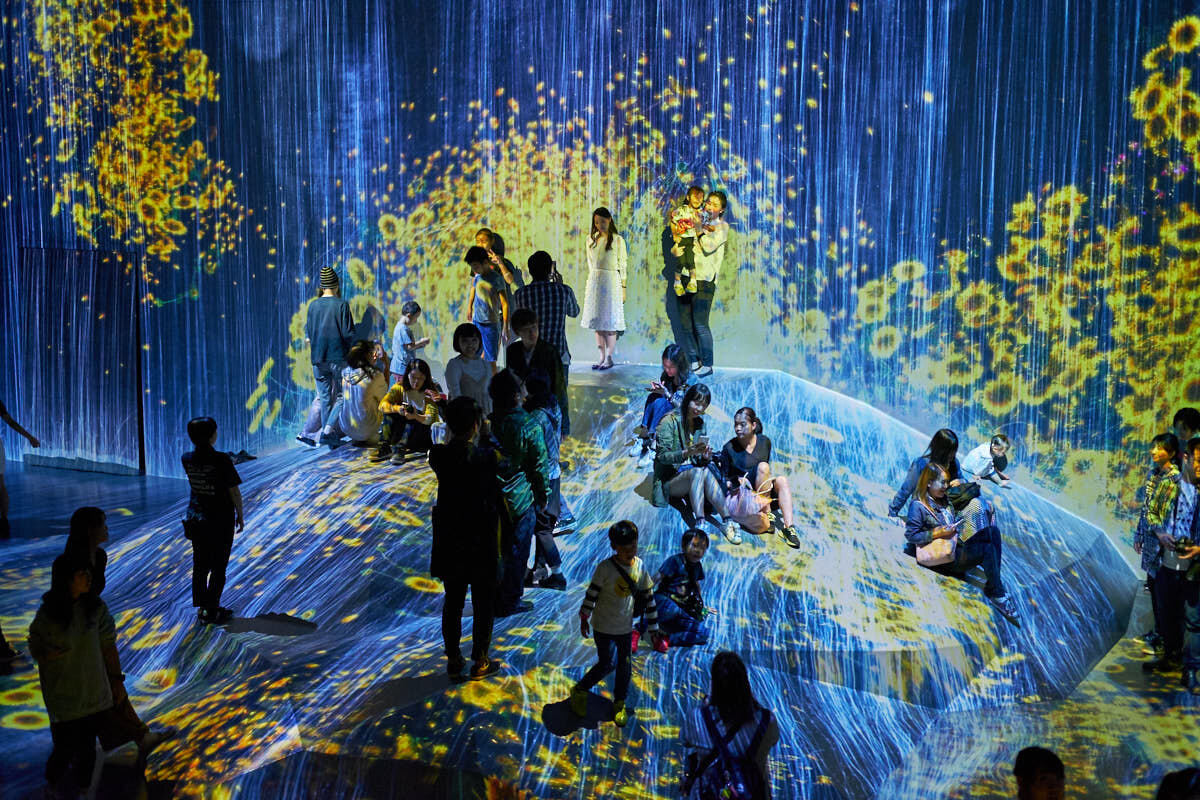The vibrant, full-color photograph captures an engaging indoor scene at an entertainment event, possibly an interactive exhibit in an Asian country. The square image is dominated by a radiant blue background adorned with projections of numerous yellow sunflowers, creating a lively, animated atmosphere. Centrally, there's a physical mound or boulder-like structure, providing a playful, elevated space. Around and atop this mound, one can see several dozen people, including families with young children. The crowd, predominantly of Asian descent, is depicted in various activities—some are standing, others sitting or relaxing, while a few take pictures, contributing to a joyful and dynamic ambiance. The clear image quality, enhanced by bright natural light, highlights the cheerful and positive environment.